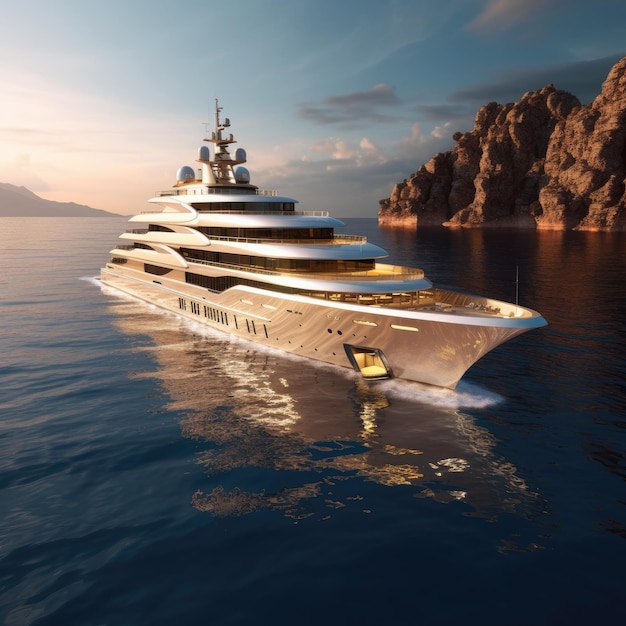This image depicts a sleek, silver, multi-story luxury yacht, possibly computer-generated. The yacht, with its five visible decks, boasts a shiny exterior that reflects the sunlight. On the top deck, there is a radar array and several spherical structures. The yacht is positioned in calm, blue waters, with its right side turned slightly toward the viewer, creating a perfect reflection on the serene surface. To the right of the vessel, there is a large rocky outcropping or island, and further in the background, a hill is visible under a light blue sky. The scene appears peaceful and devoid of any people, animals, or additional structures, emphasizing the yacht's solitary grandeur in this idyllic setting.